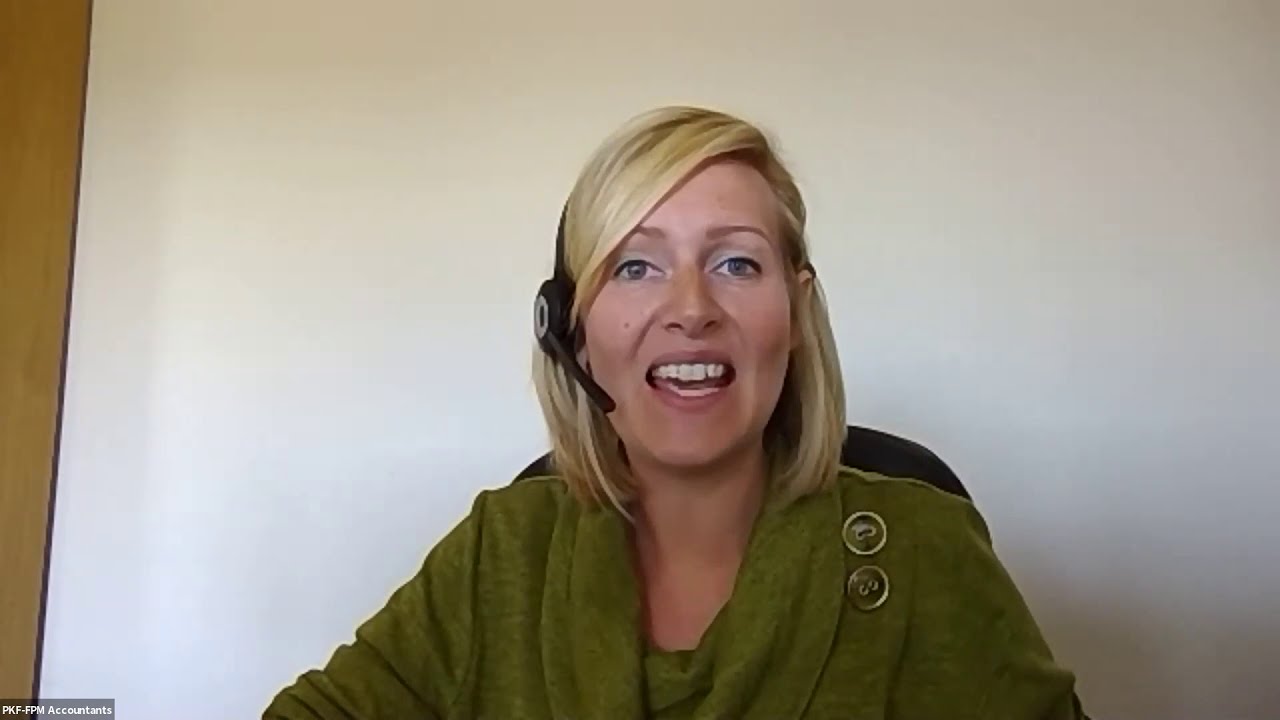A blond-haired woman with shoulder-length hair parted on the side and bangs sweeping across her face is captured looking directly into the camera. Her mouth is open, revealing her white teeth, as she speaks into a black headset. The woman, who has light-colored eyeshadow and possibly gray eyes, is sitting in a black chair against a predominantly white wall with a sliver of a brown section to the far left of the image. She is wearing an olive green cowl-neck sweater adorned with two large buttons of the same color on the upper left side. The image, taken from the chest up, includes small white text on the bottom left corner that reads "PKF-FPM Accountants."